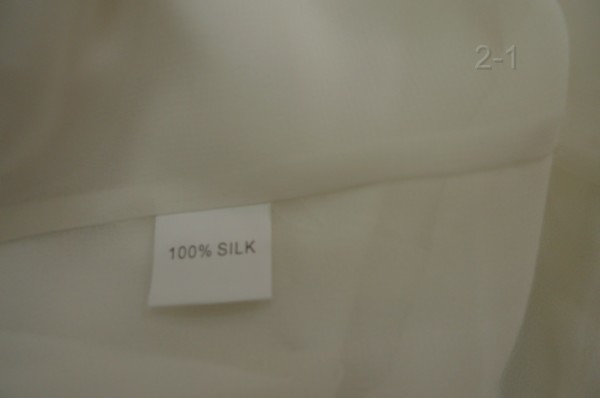The image displays a real photograph of a piece of fabric against a grayish background, appearing slightly shadowed and slightly out of focus. Extending from the left side to about five-sixths of the way to the right, the fabric has a white hue with a darker portion at the top. A notable seam runs horizontally across the fabric, creating an upper and lower section. In the upper right corner, the numbers "2-1" are visible, seemingly embroidered or digitally added. Beneath the seam, a white tag with black text reads "100% silk." The fabric appears darker due to shadowing, suggesting the photograph was taken in a dimly lit room.